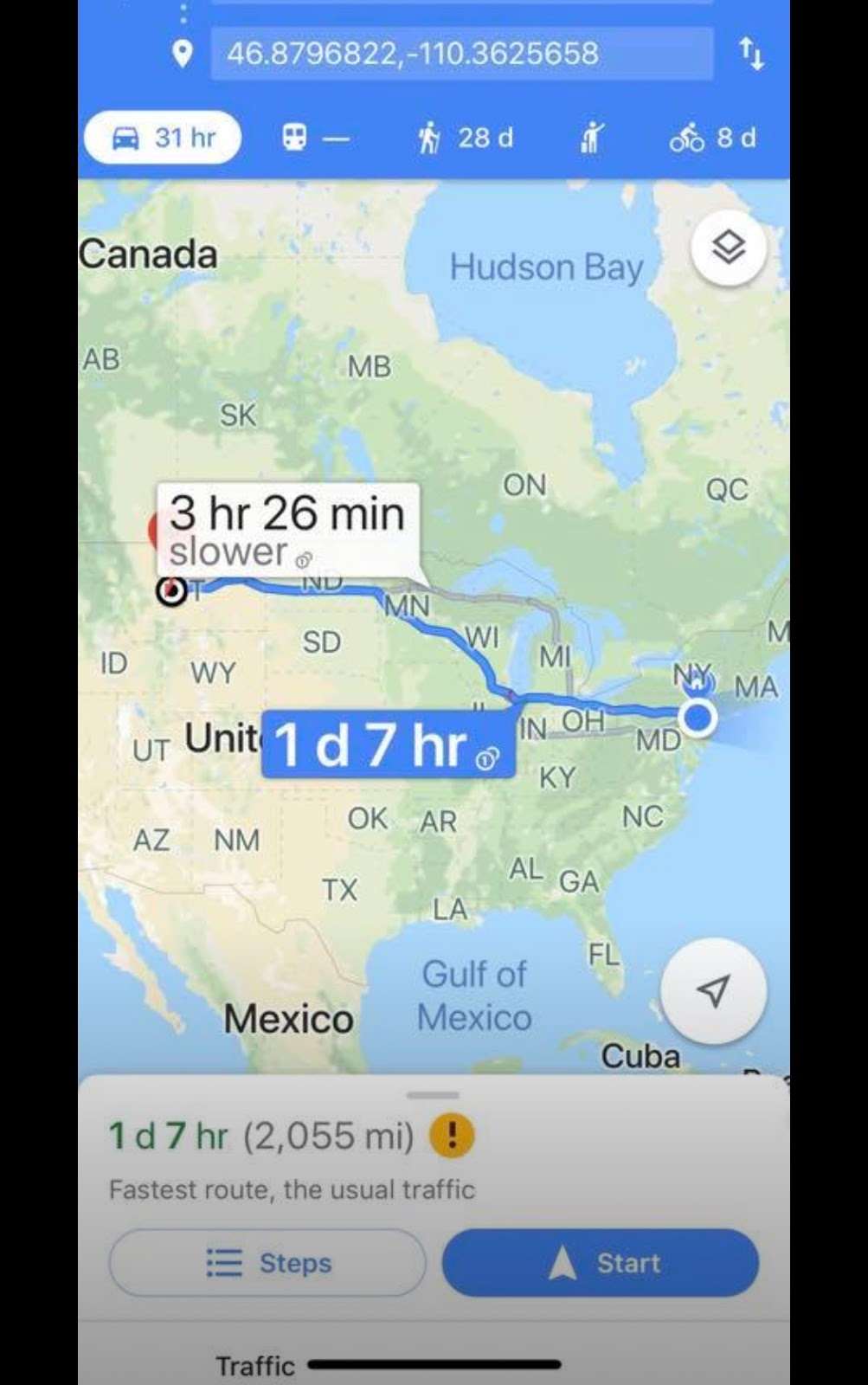Here is a cleaned-up and detailed description of the image:

---

This image, seemingly captured from a phone, appears to be a screenshot of a navigation app or GPS display. The screen shows a portion of a route planning interface, albeit slightly cut off at the top, with prominent black bars on either side of the image. 

At the top left, partially visible coordinates (46.8796822,-110.3625658) are displayed, suggesting the destination location. Next to it on the right, there's an option to reverse the directions, although the starting point is not visible due to the cutoff.

Beneath this, several transportation options are depicted. Highlighted is a car icon with an estimated travel time of 31 hours. Additional icons include:
- A plane symbol (travel time not specified in the description).
- A walking icon indicating a travel time of 28 days.
- An unknown symbol of a person holding what seems like a suitcase.
- A bicycle icon with a travel time of eight days.

The bulk of the screen showcases a map focusing mainly on the United States, including glimpses of Canada to the north and Mexico to the south. The starting point appears to be somewhere between New York and Maryland, with the route extending east to west across the United States. The destination is shown to be somewhere west of the Dakotas, possibly between Idaho and Wyoming, though the exact location is obscured.

On the route, a white box indicates "3 hours, 26 minutes slower," referring to an alternative path. The primary route, marked in blue, displays a travel time of "1 day, 7 hours" in both a blue and a white box, clarifying that the total distance is 2,055 miles.

---

This description provides a comprehensive overview of the image, detailing the navigation app's interface and the specifics of the route displayed.